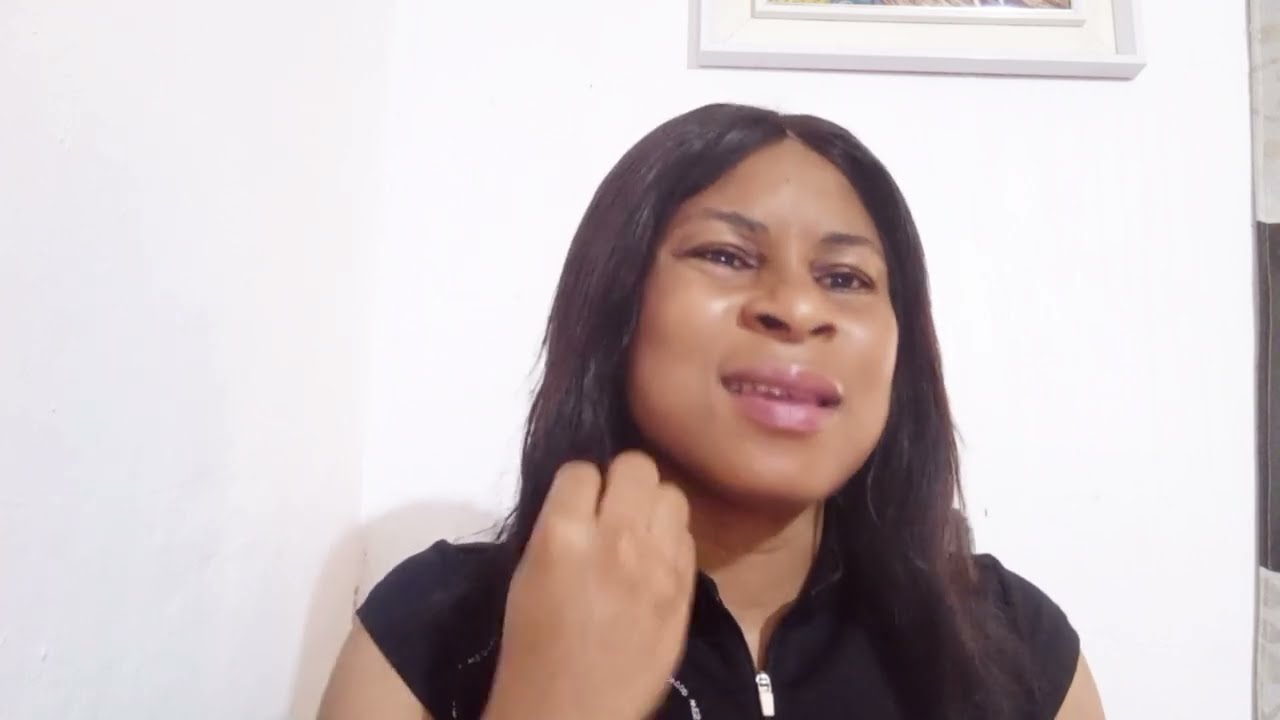The image depicts a black woman with dark skin, shoulder-length straight hair parted down the middle, and dark eyes. She is wearing a black top with cap sleeves and a silver zipper down the middle. Her lips are adorned with pink lip gloss, and her right hand is raised near her right cheek while her mouth is slightly open, revealing the top row of her teeth, as if she is speaking or explaining something. The background is a stark white wall with a partially visible white picture frame in the upper right corner and possibly a curtain with sections in white and gray to the far right. The woman appears to be in her early 30s and is looking directly at the camera with an expression that suggests engagement or conversation.